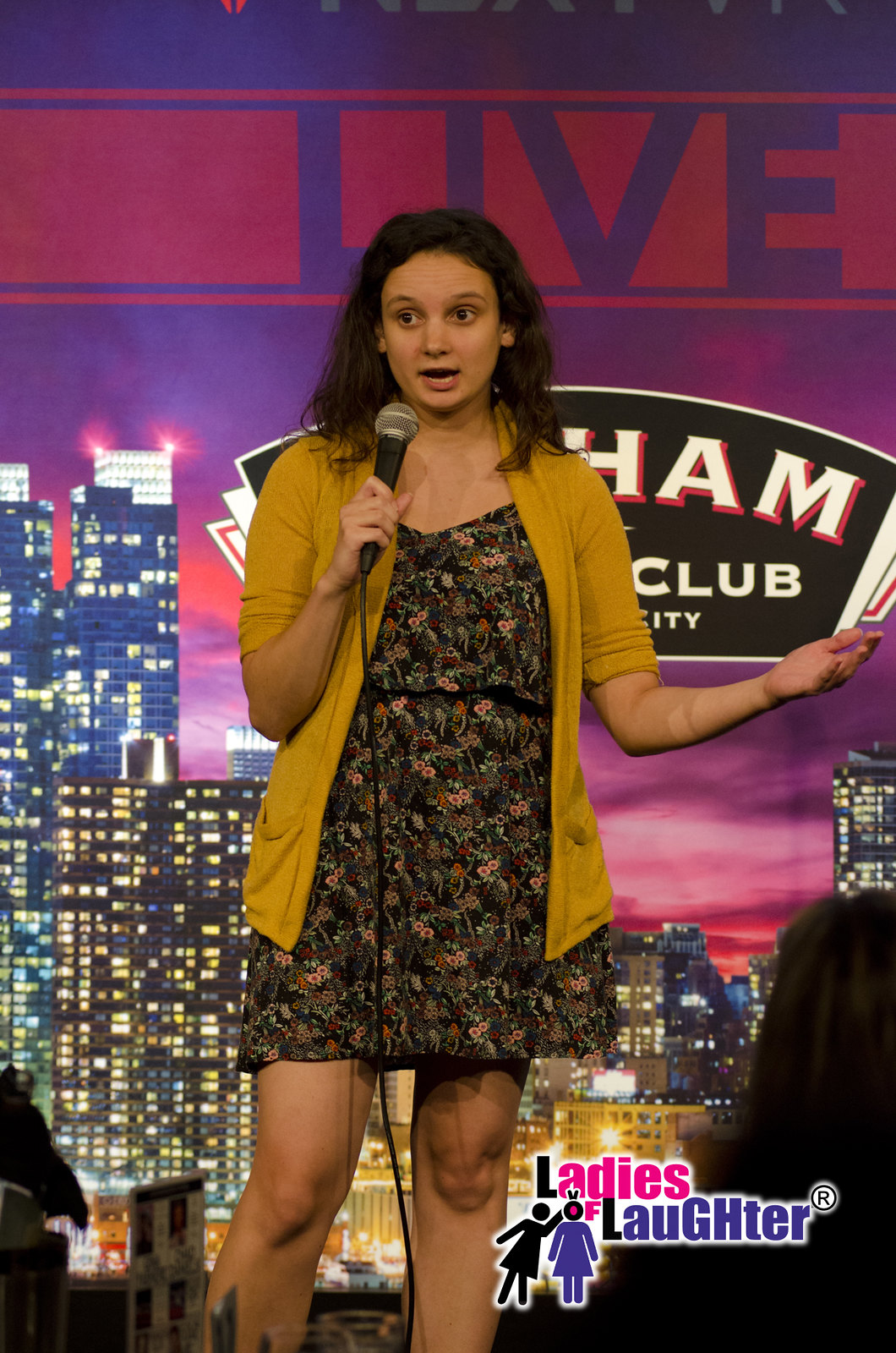This is an image of a woman, likely in her mid to late twenties, holding a microphone on a stage, possibly captured from a photograph or video screen grab. She stands in front of a vibrant, illuminated cityscape mural, showcasing an array of skyscrapers and apartment buildings at night. The backdrop prominently features the word "LIVE" in blue against a red background, along with partially obscured letters ending in "H-A-M" followed by "Club City," suggesting a comedy venue or event location. A watermark in the lower right corner reads "Ladies of Laughter" in pink and purple, indicating that this is most likely a comedy performance.

The comedian is a white woman with shoulder-length dark hair left loose. She is dressed in a black dress adorned with pinkish floral prints and a yellow cardigan. She holds the microphone in her right hand while gesturing expressively with her left hand, palm up, as if she's mid-joke or storytelling. Her mouth is open, and she appears to be addressing the audience, fully engaged in her performance.